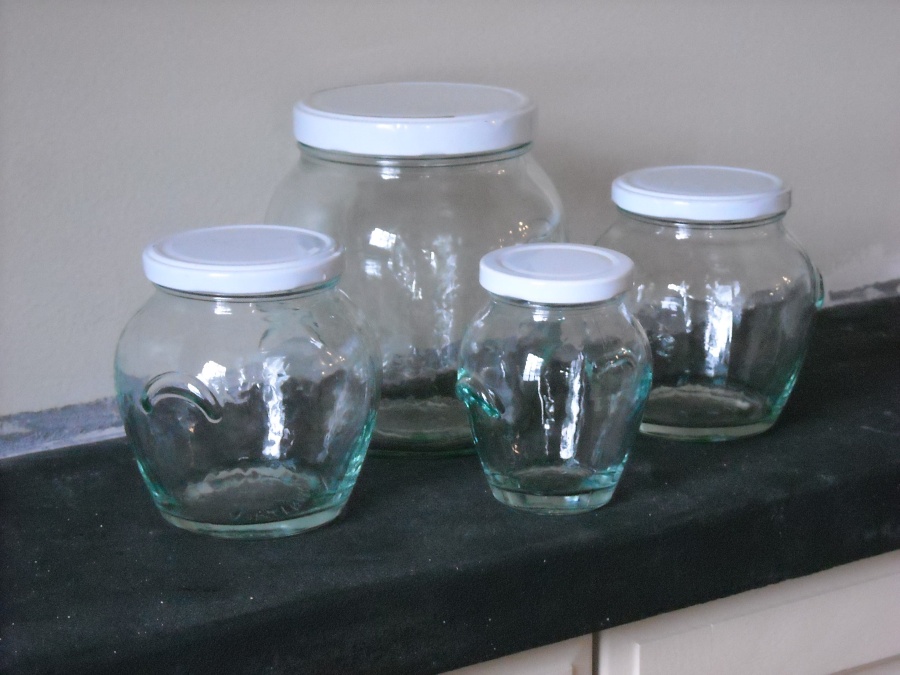This image showcases an indoor setting featuring four transparent glass jars of different sizes, all with white twist-on lids. The jars are placed on a black countertop that appears to curve slightly. The background consists of a white or light gray wall and white wooden cabinets below the countertop. The countertop itself seems to be covered with a white, dusty substance. 

Arranged in an almost symmetrical pattern, the jars are set in front of the wall: the largest jar is positioned at the back left, while a slightly smaller jar is at the back right. In the front, a large jar sits to the left of a smaller jar positioned at the front right. The glass jars have a unique design, featuring flared tops that curve outward before tapering into flat bottoms. A distinctive crescent or sideways banana shape can be observed on their surfaces. The jars are empty, containing no liquid or objects.